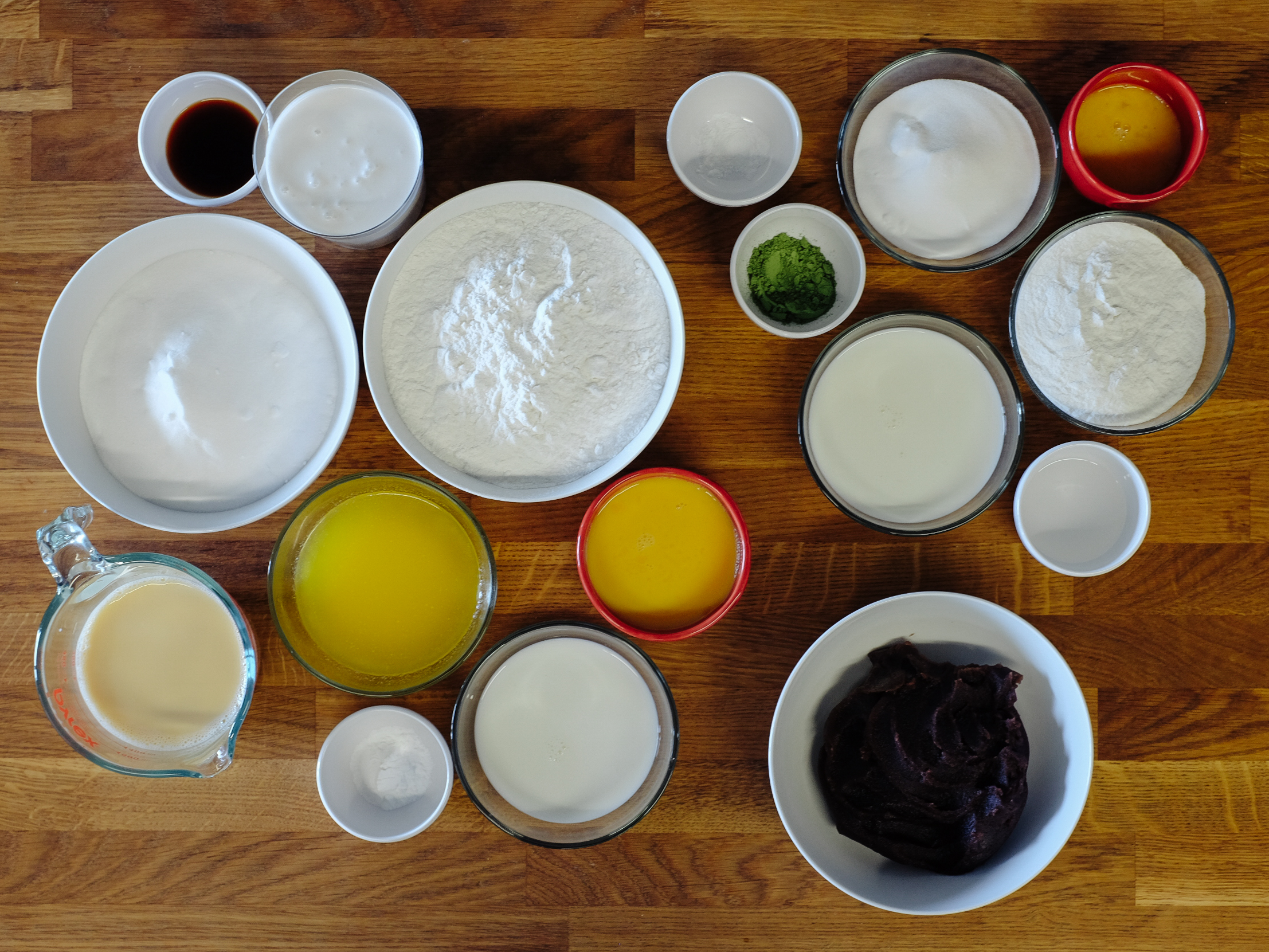This horizontal, top-down photograph captures a variety of bowls of different sizes and colors arranged on a wooden table, each containing pre-measured ingredients likely for a recipe preparation. The collection includes white ceramic bowls filled with powders that might be different types of flour or sugar, and a few bowls with creamy or broth-like yellow liquids. There's a Pyrex measuring cup with a cream-colored liquid that could be buttermilk or cream. Other noteworthy elements include a small white bowl with a green substance, possibly chives or another finely chopped vegetable, and another bowl with a dark substance, maybe cranberry sauce or date paste. Additionally, there are several red plastic bowls, some larger and some medium-sized clear glass and orange bowls. Among these, there is a dark reddish-black liquid, likely soy sauce or a concentrated spice mixture, and a very dark, almost black paste that resembles tar or jello. The preparation appears intricate, with various stages of the cooking process laid out across the wooden surface.